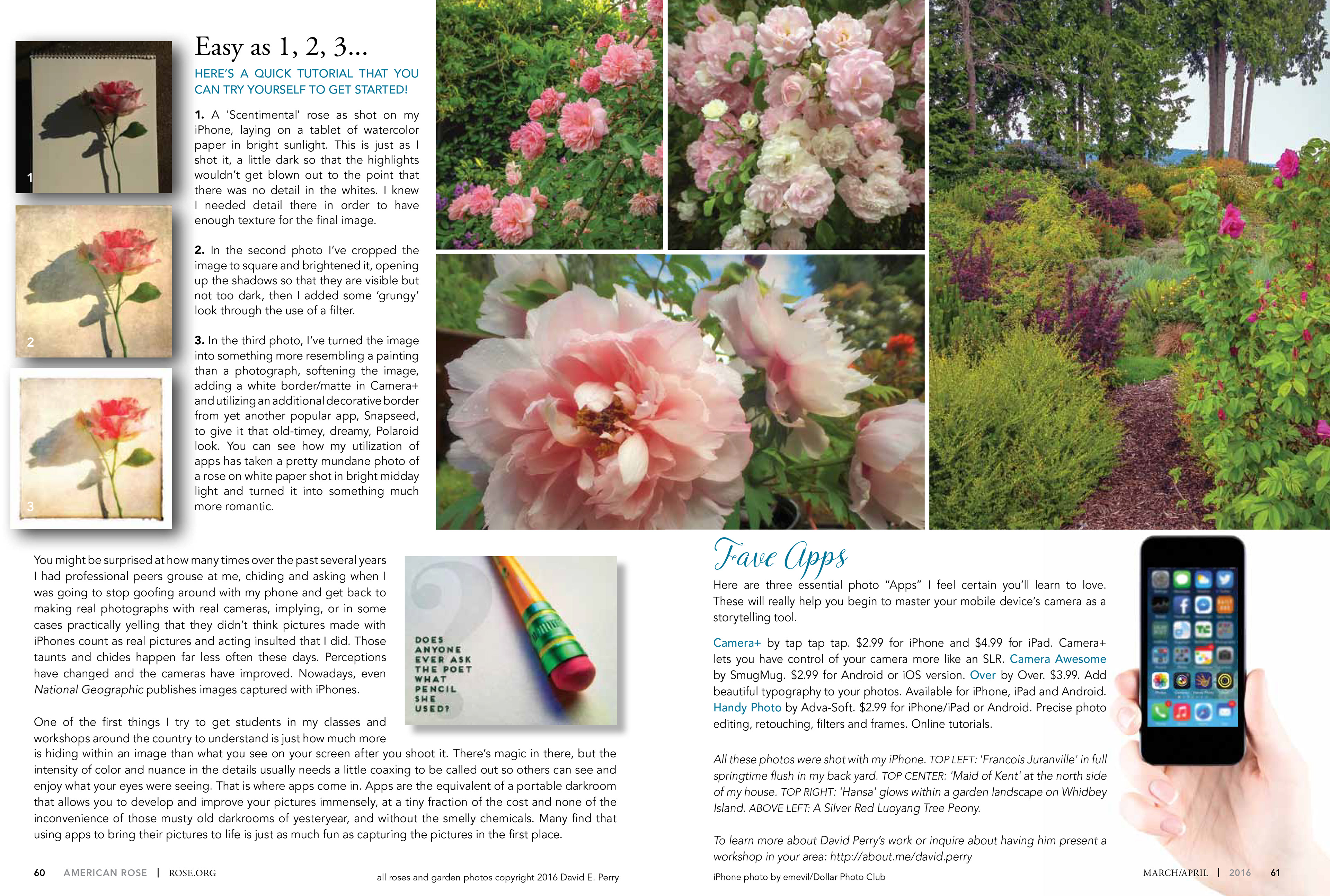The advertisement, titled "Easy as 1, 2, 3," features a vibrant and colorful visualization with a mix of photographic and illustrative elements laid out across what appears to be a two-page magazine spread. Central to the image is a black phone held by either a man or woman, displaying multiple screenshots of favorite apps. The ad is designed as a tutorial for using these apps to photograph flowers, featuring text that is lengthy but small and somewhat difficult to read.

Flanking the phone are detailed floral visuals. On the left side, there are three individual images of flowers ranging in colors from pink to red, set against lush green foliage with hints of purple on the outer edges. The right side similarly showcases three or four images depicting gardens and forest scenes filled with vibrant flowers.

The text in the ad includes various statements like "written in blue" and “Fade Apps in blue,” highlighting the tutorial nature of the advertisement. Additional details like a little pencil icon suggest an emphasis on photo editing. There’s also a note about the pages within the magazine: page 60 on the right containing three drawn images of a rose in different lighting conditions, and page 61 on the left featuring actual photographs of roses. Accompanying these images are various copyrights and additional text, providing an informative background on the content.

Overall, this detailed ad blends technology and nature, showcasing an app's capability to capture and enhance the beauty of flowers, all while being easy to use, as indicated by the prominent "Easy as 1, 2, 3" slogan.